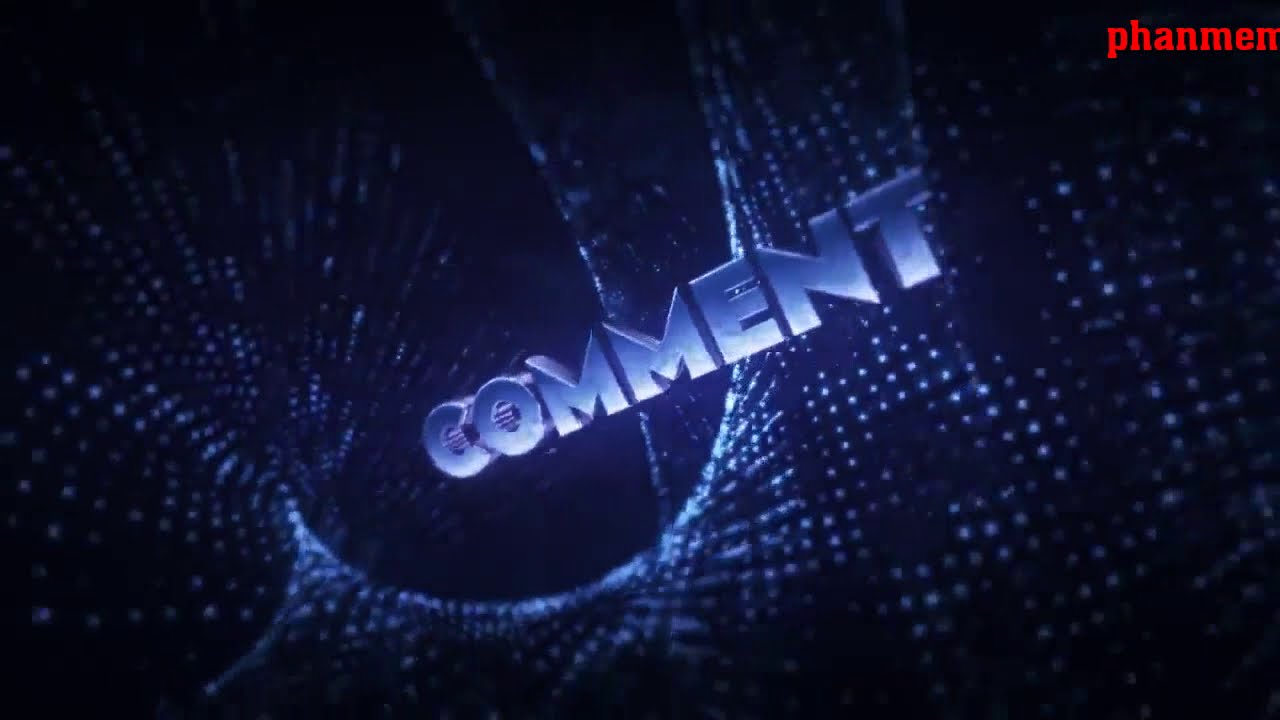The digital image features a visually striking graphic design set against a dark purple to black gradient background, adorned with a web-like pattern and clusters of white and blue dots. These dots create a shimmering, almost animated texture that twists and funnels towards the left side of the image. Dominating the center of the composition is the word "COMMENT," spelled out in bold, capital 3D letters that gradually shift in color from whitish at the bottom to a dark purplish-blue at the top. This text is oriented diagonally, ascending from the center-left towards the upper-right corner of the frame. In the top-right corner, partially obscured by the design, are red lowercase letters spelling out "phanmen" or "fun namen." The entire image has a dynamic and engaging feel, reminiscent of digital posters or screen stills encouraging viewer interaction, typical of YouTube or social media prompts.